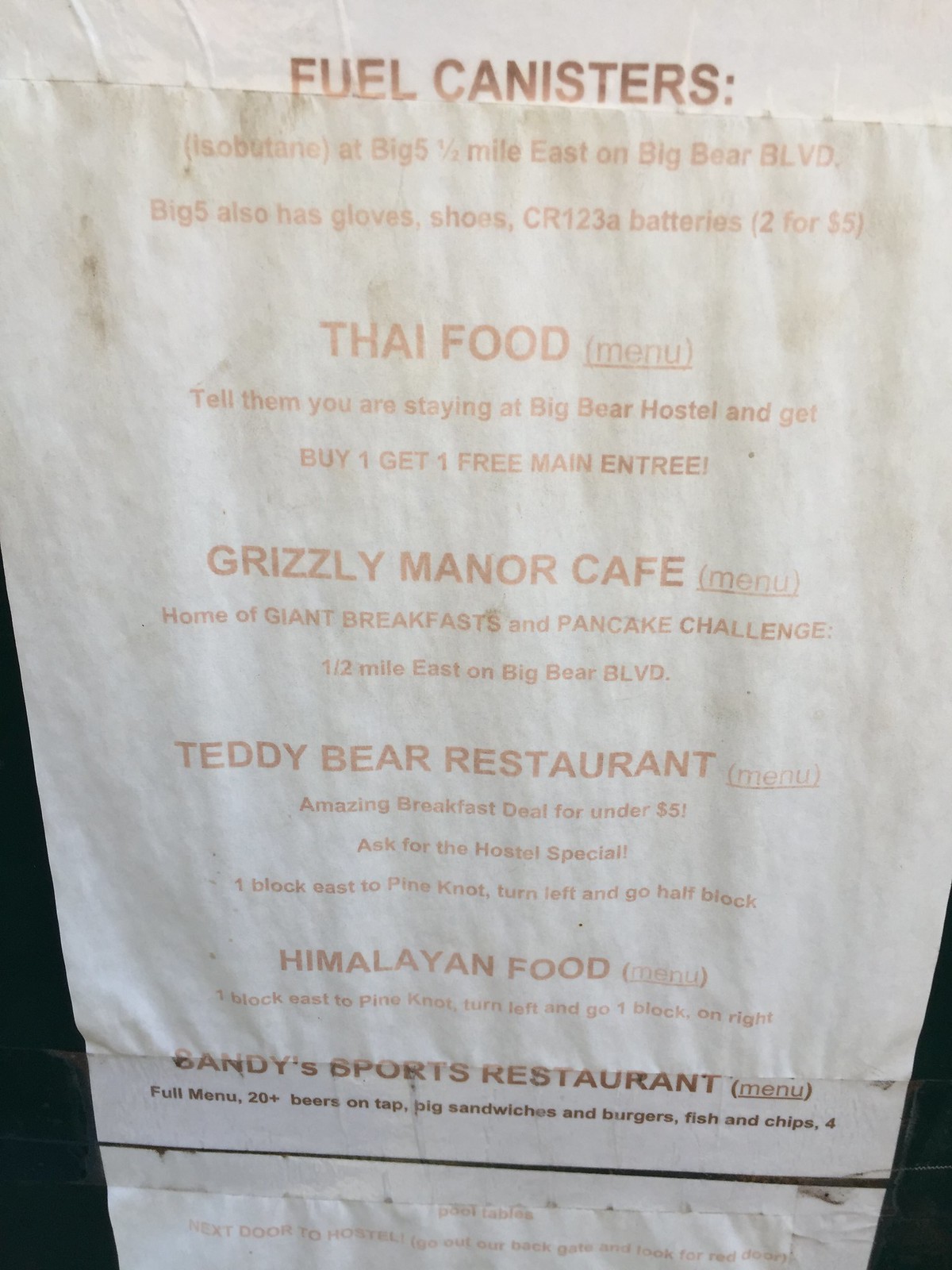A faded poster, appearing to have been taped to a door, serves as a guide for local amenities and attractions around Big Bear Boulevard. At the top, in what used to be maroon-colored, bold letters, the heading "Fuel Canisters" stands out, although now considerably faded to a maroonish-brown. Underneath, various items and services are listed with detailed directions:

- **Fuel Canisters**:
  - **Isobutane**: Available at Big Five, located five and a half miles east on Big Bear Boulevard. Big Five also stocks gloves, shoes, and CR123A batteries, priced at two for five dollars.

- **Thai Food**:
  - To avail of a buy one get one free main entrée offer, inform them you are staying at Big Bear Hostel.

- **Grizzly Manor Cafe**:
  - Noted for its giant breakfast and pancake challenge, situated half a mile east on Big Bear Boulevard (abbreviated as BLVD in regular typeface).

- **Teddy Bear Restaurant**:
  - Offers an amazing breakfast deal for under five dollars. Request the hostel special. It's located one block east to Pine Knot, turn left, then go half a block.

- **Himalayan Food**:
  - Found one block east to Pine Knot, turn left and proceed one more block on the right.

- **Sandy’s Sports Restaurant**:
  - Features a full menu with over 20 beers on tap, big sandwiches and burgers, as well as fish and chips.

A partially covered second paper peeks from underneath, providing further details about Sandy’s Sports Bar and additional amenities:
  - Pool tables next door to the hostel. Exit through the back gate and look for the red door. 

This poster appears to be a helpful resource for hostel guests and local explorers, detailing the various food and drink options, with clear directions for easy navigation.